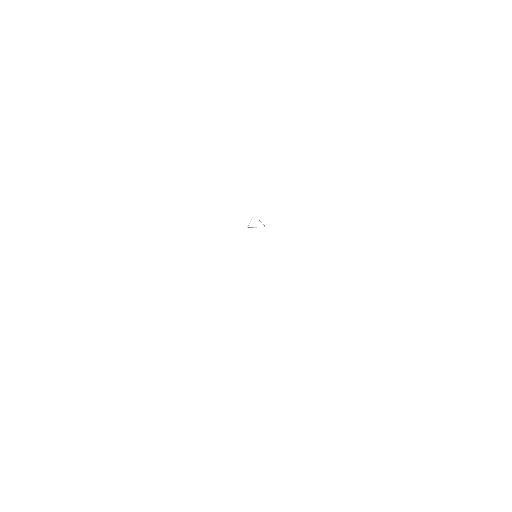The image prominently features a minimalistic design on an otherwise empty, predominantly white background. Centrally placed is a minuscule graphic, approximately 4 to 5 centimeters in size, depicting what appears to be an open book or a notebook outlined in black. A faint line runs through the center of this tiny illustration, adding to its enigmatic nature. The overall impression is reminiscent of a placeholder icon for broken or missing images frequently seen on websites. Devoid of other elements, the strikingly small and ambiguous notebook accompanied by the line creates a curious focal point amidst the vast whiteness, leading one to ponder its purpose and origin.